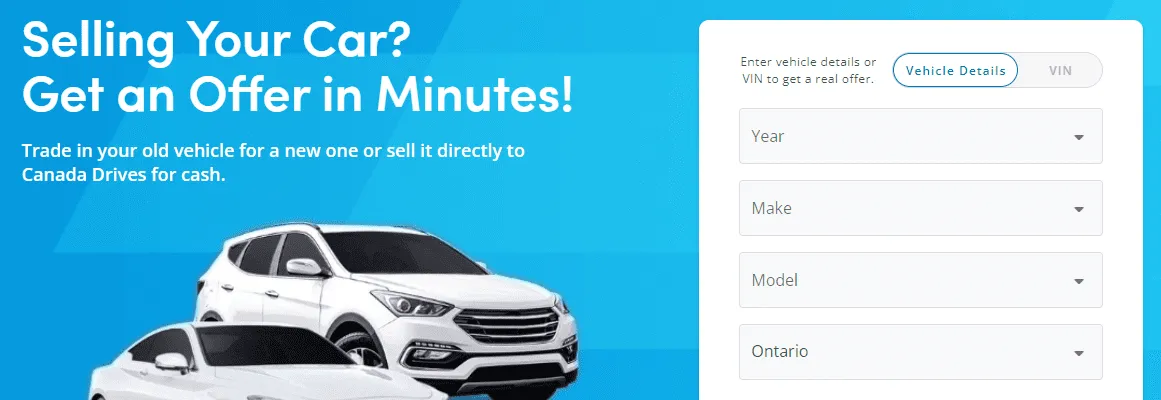The image showcases a simple and efficient process for selling your car. With the option to get an offer in minutes, you can either trade in your old vehicle for a new one or sell it directly to Canada Drives for cash. To receive a genuine offer, you need to enter your vehicle details or Vehicle Identification Number (VIN), including information such as the year, make, model, and location—in this case, Ontario. The visual features a sleek design with a white and blue color scheme, highlighting two automobiles: a white SUV and a white sedan, representing the types of vehicles you can trade or sell through this service.